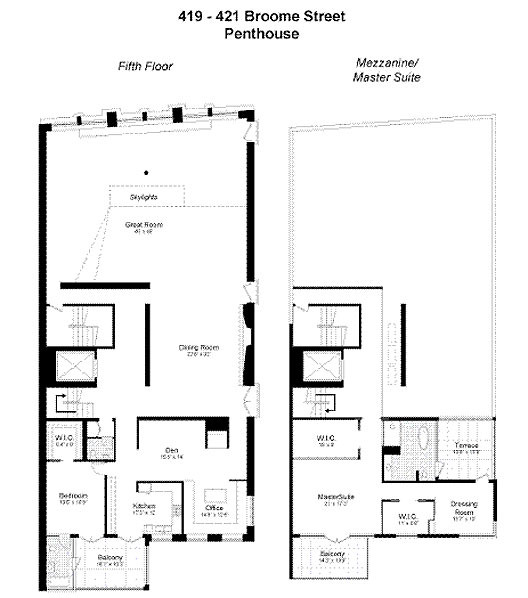The image showcases the floor plans of a penthouse located at 419-421 Broom Street with detailed layouts for two separate levels. At the top of the image, the title "419-421 Broom Street Penthouse" is prominently displayed.

On the left side, the floor plan for the 5th floor is presented. This floor is structured as a giant rectangle with various rooms labeled, though some labels are difficult to discern due to the blurriness and distant perspective of the screenshot. Notably, the top right section of this floor plan is designated as the dining room. Adjacent to it on the left, a staircase is depicted, indicating access to other levels. Additional rooms identified on this floor include an office situated at the bottom right, a bathroom at the bottom left, and a space possibly labeled as a gallery or bakery at the very bottom, though the text is unclear.

On the right side of the image, the floor plan for the Mezzanine Master Suite is displayed. This floor plan indicates a spacious master suite occupying the top section, with no specific rooms labeled in that area. However, distinct rooms listed on this floor include a bathroom, a dressing room, and a space labeled "WIC," the meaning of which is unclear. Another area on this floor plan appears to be labeled "Masa Duke," though the text is barely legible due to the image's low resolution.

Overall, the screenshot attempts to convey a detailed layout of the penthouse's 5th floor and mezzanine level, though the quality of the image makes precise identification of some areas challenging.